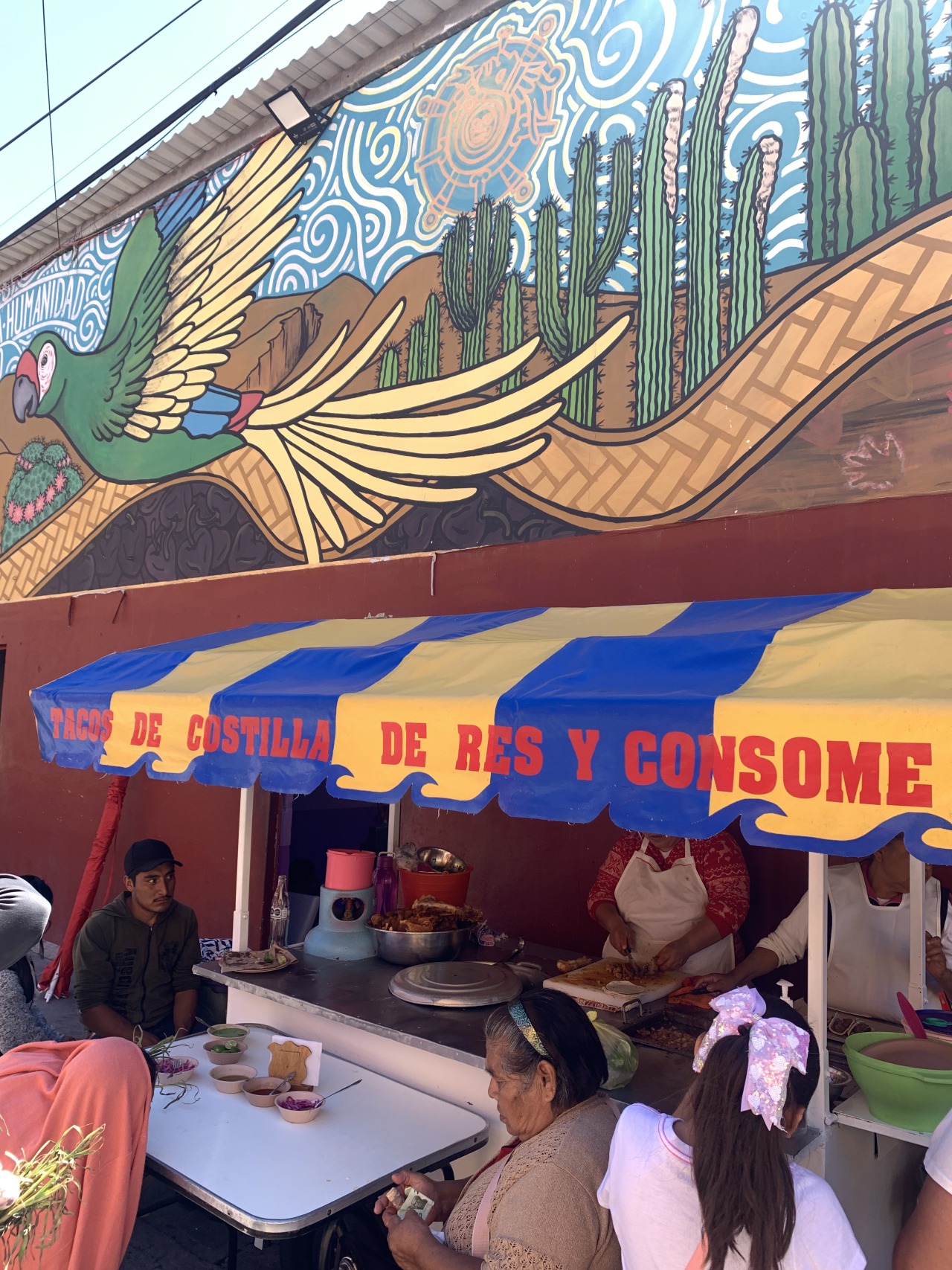This photograph depicts a vibrant street-side restaurant with a distinctive blue and white awning featuring red text that reads "tacos de costilla de res y consome." Beneath the awning, two workers are diligently preparing food. The worker on the right, in a red top and white apron, is focused on chopping meat on a white cutting board. To their left, another worker in a white long sleeve shirt and apron is also engaged in food preparation. 

In the foreground, a woman with a headband sits at an outdoor table, concentrating on an item in her hands. Across from her, a man in a baseball cap and dark top peers into the kitchen area. Behind this seated woman, another lady with long dark hair, a pink bow, and a light-colored t-shirt is partially visible, along with the shoulder of a person beside her. 

The upper part of the image is adorned with a mural depicting a green parrot with yellow and blue-tipped wings soaring across a desert landscape filled with cacti. The sky within the mural is artistically decorated with white swirls and an intricately designed sun. Brown gutters and a compact arrangement of about six bowls of food on the table accentuate the lively, intimate atmosphere of this bustling eatery.